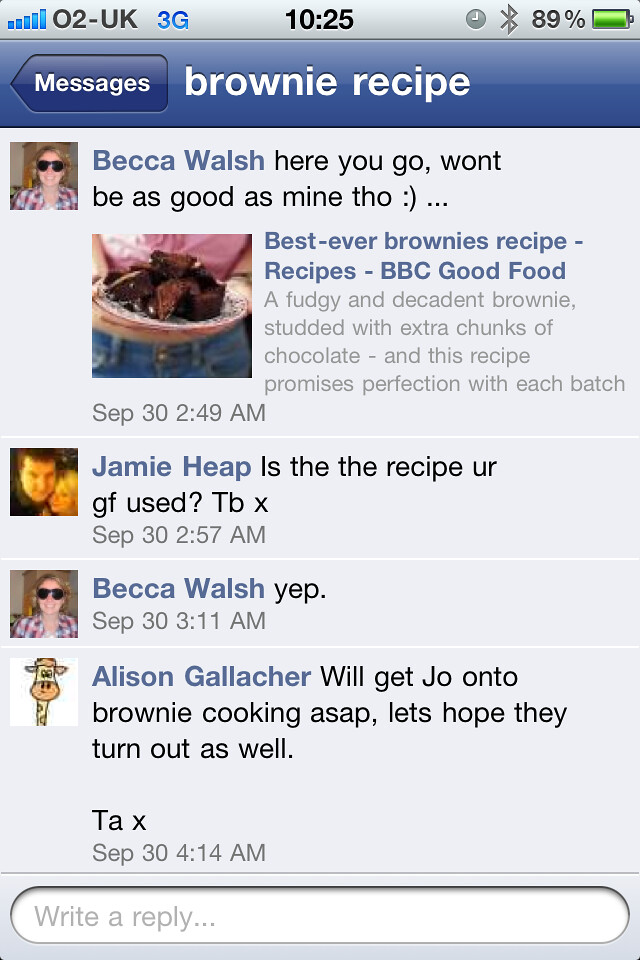This is a detailed screenshot of an old iPhone messaging screen set in the UK, as indicated by the "O2 UK" carrier and "3G" network status. The time on the phone shows 10:25 with the battery at 89%. The conversation involves multiple people, namely Becca Walsh, Jamie Heap, and Allison Gallagher, discussing a brownie recipe. Becca Walsh starts by sharing a recipe titled "Best Ever Brownies Recipe" from BBC Good Food along with a message, "Here you go, won't be as good as mine though." Below her message, there's a picture of a woman holding a plate of mini brownies and a detailed recipe description: "A fudgy and decadent brownie studded with extra chunks of chocolate. This recipe promises perfection with each batch," dated September 30th at 2:49 AM. Jamie Heap responds, asking, "Is this the recipe your girlfriend used?" at 2:57 AM. Allison Gallagher then chimes in, expressing enthusiasm, "We will get you onto brownie cooking ASAP. Let's hope they turn out well." The entire exchange takes place on a classic bluish-gray iPhone interface, adding a nostalgic touch to the visual.